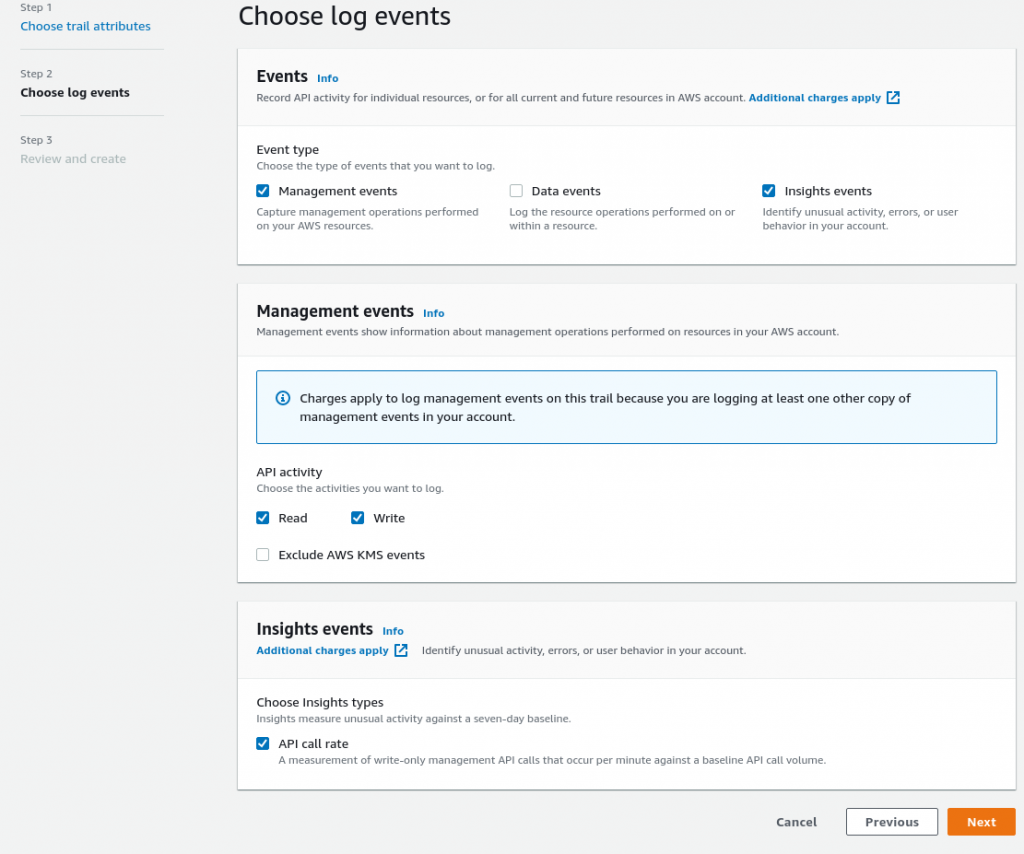This screenshot captures the settings interface of an Amazon Web Services (AWS) setup, characterized by a predominantly gray background. The interface is part of the process for configuring logging events for a trail, as suggested by the color scheme, font choices, and button placements typical of AWS applications.

On the left-hand side, there is a step-wise guide for setting up the trail:
- **Step 1**: Choose Trail Attributes
- **Step 2**: Choose Log Events
- **Step 3**: Review and Create (currently grayed out, indicating it is not accessible yet)

The top middle section features the heading **"Choose Log Events"**, followed by detailed instructions:
- **"Events Info"**: Record API Activity for Individual Resources or for All Current and Future Resources in your AWS Account (noting that additional charges may apply)
- **"Event Type"**: Choose the type of events you want to log

Below this heading are various options with corresponding checkboxes:
- **Management Events**: (Checked) - Captures management operations performed on your AWS resources.
- **Data Events**: (Unchecked) - Logs the resource operations performed on or within a resource.
- **Insights Events**: (Checked) - Identifies unusual activity, errors, or user behavior in your account.

Further down, there is additional information under a second **"Management Events Info"** section, explaining that management events show details about management operations carried out on resources within the AWS account. A blue, rectangular warning box indicates that charges apply for logging management events in this trail because at least one other copy of management events is being logged in the account.

Following this, under **"API Activity"**, users can choose specific activities to log. The options available include:
- **Read/Write**: (Checked)
- **Exclude AWS KMS Events**: (Unchecked)

At the bottom of the interface are navigation buttons:
- **Cancel**
- **Previous**
- **Next**

These buttons allow users to navigate through the setup steps, cancel the configuration, or proceed to the next stage.